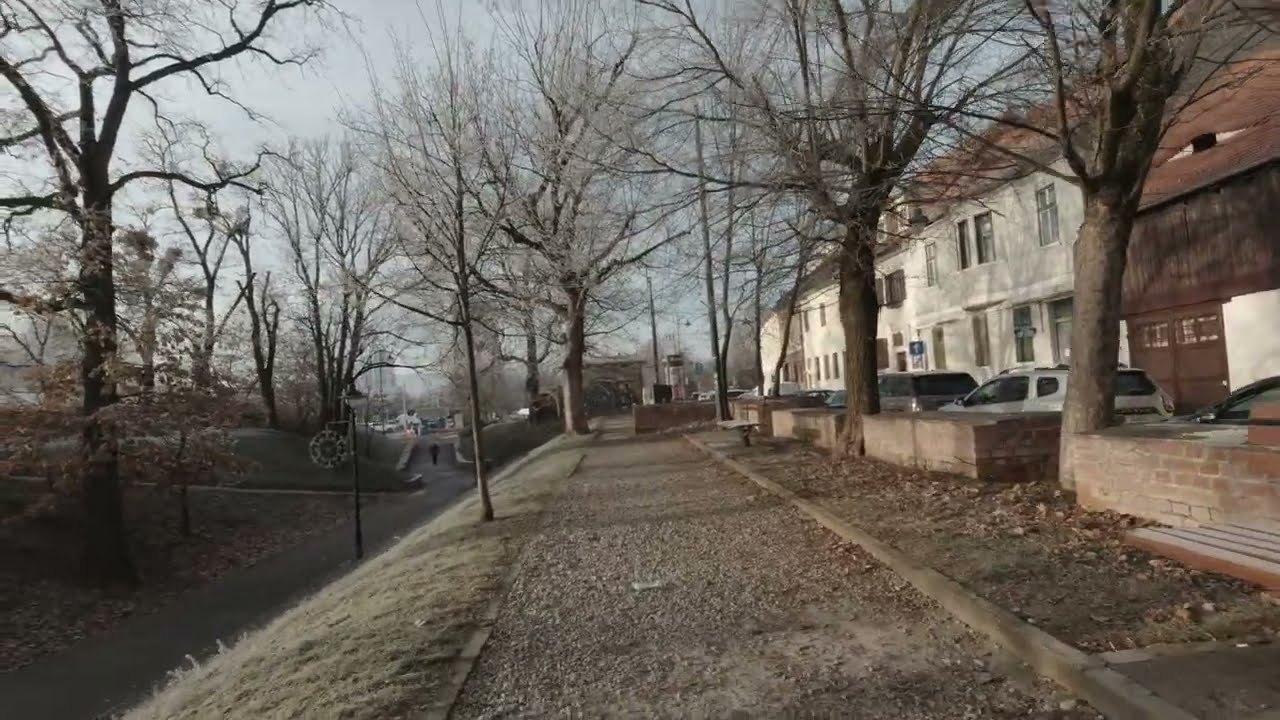The image depicts a small townscape during winter, indicated by the bare trees devoid of leaves. A slightly worn gravel pathway runs through the center of the image, flanked by cement or wood borders. The path appears to be adjacent to a street or parking area, as several cars are visible parked beside white and brown buildings with terracotta roofs and brick structures or planting boxes. On both sides of the path, there are large, leafless trees lining the way, contributing to a stark, wintry atmosphere. To the left of the gravel walkway, a grassy slope descends to another pathway, where a person dressed in black is seen walking or running in the distance. The scene includes additional urban elements such as a light brown bench with a touch of frost and dotted streetlights. The sky overhead is predominantly gray, enhancing the subdued winter setting. Overall, the image captures a tranquil yet slightly desolate urban park area interwoven with residential and possibly commercial buildings.